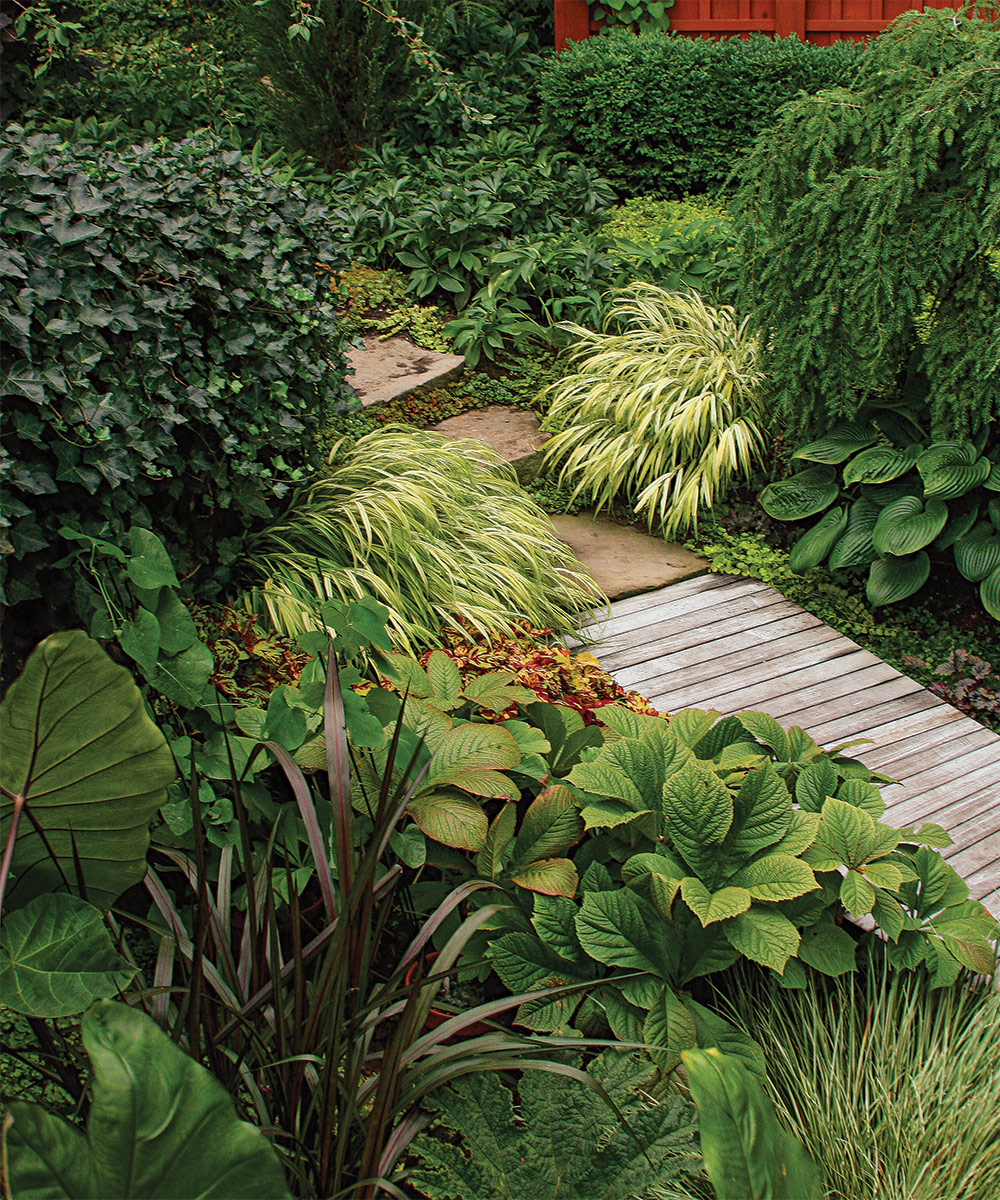This photograph captures a richly detailed garden pathway. The path, starting at the lower right and extending diagonally to the upper left, features a combination of light gray wooden planks and large brown flagstones. The wooden walkway transitions into a series of stone slabs that make up the rest of the path. On both sides of the pathway, a diverse array of plants flourishes, ranging from short ground cover to waist-high bushes in various shades of green, yellow, red, and even some purples. To the right, a reddish brown structure and part of a lower wall can be seen peeking through the vibrant foliage. The plants include regular garden bushes, shrubbery poised to bloom, and grassy plants with blade-like leaves, all contributing to the lush, natural scenery. Trees in the background add to the overall verdant ambiance, making it a serene snapshot of nature's beauty.